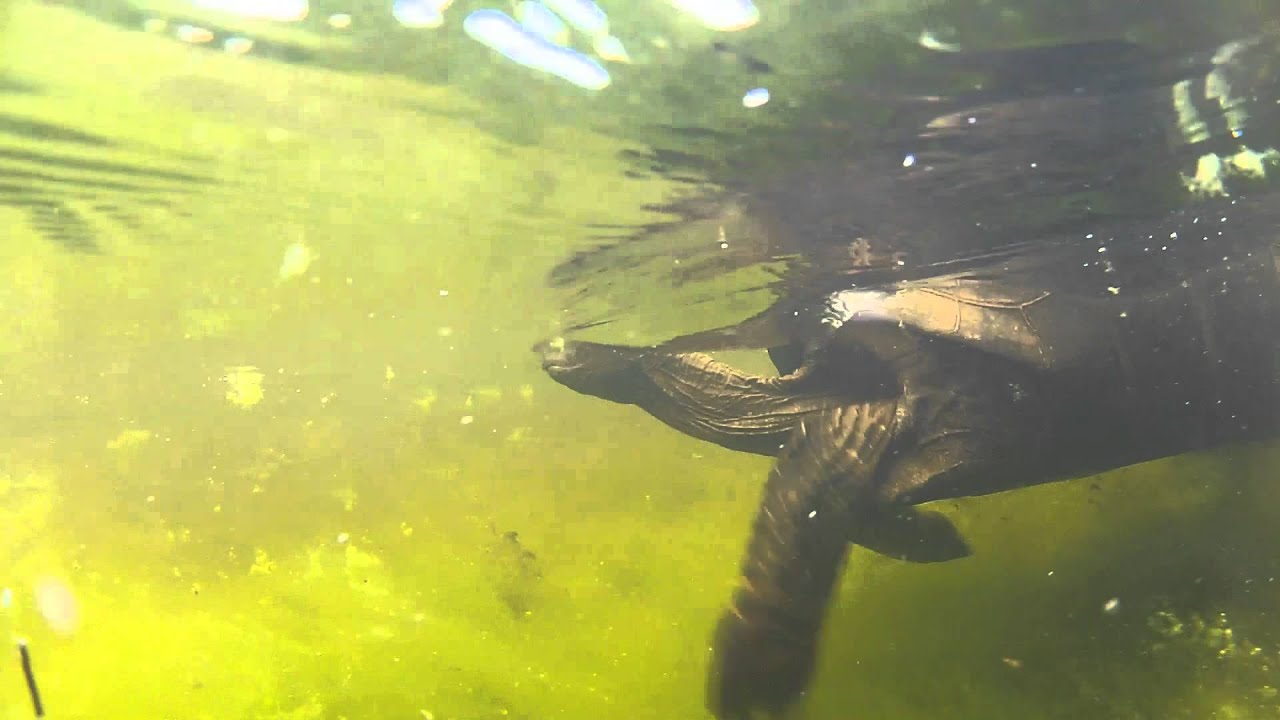In this underwater photograph, a turtle is depicted swimming just below the surface of a pond. The pond water is a murky green, filled with hazy flecks, giving it an almost lime green hue suggestive of algae. The turtle's long neck and a portion of its head extend above the water, with just the top part of its shell peeking out as well. Below the water, the turtle’s front legs, the side of its shell, and the underside are clearly visible. The turtle's shell and skin are dark olive green, providing a strong contrast to the vibrant pond water. The seafloor, adorned with blurry foliage, can be seen in the background, adding depth to the scene. Light from above the water surface and a secondary source from the lower left illuminate the turtle, highlighting its movements and casting subtle reflections. The turtle's motion creates a small wake behind it, indicating a sense of progression through this algae-filled aquatic environment.